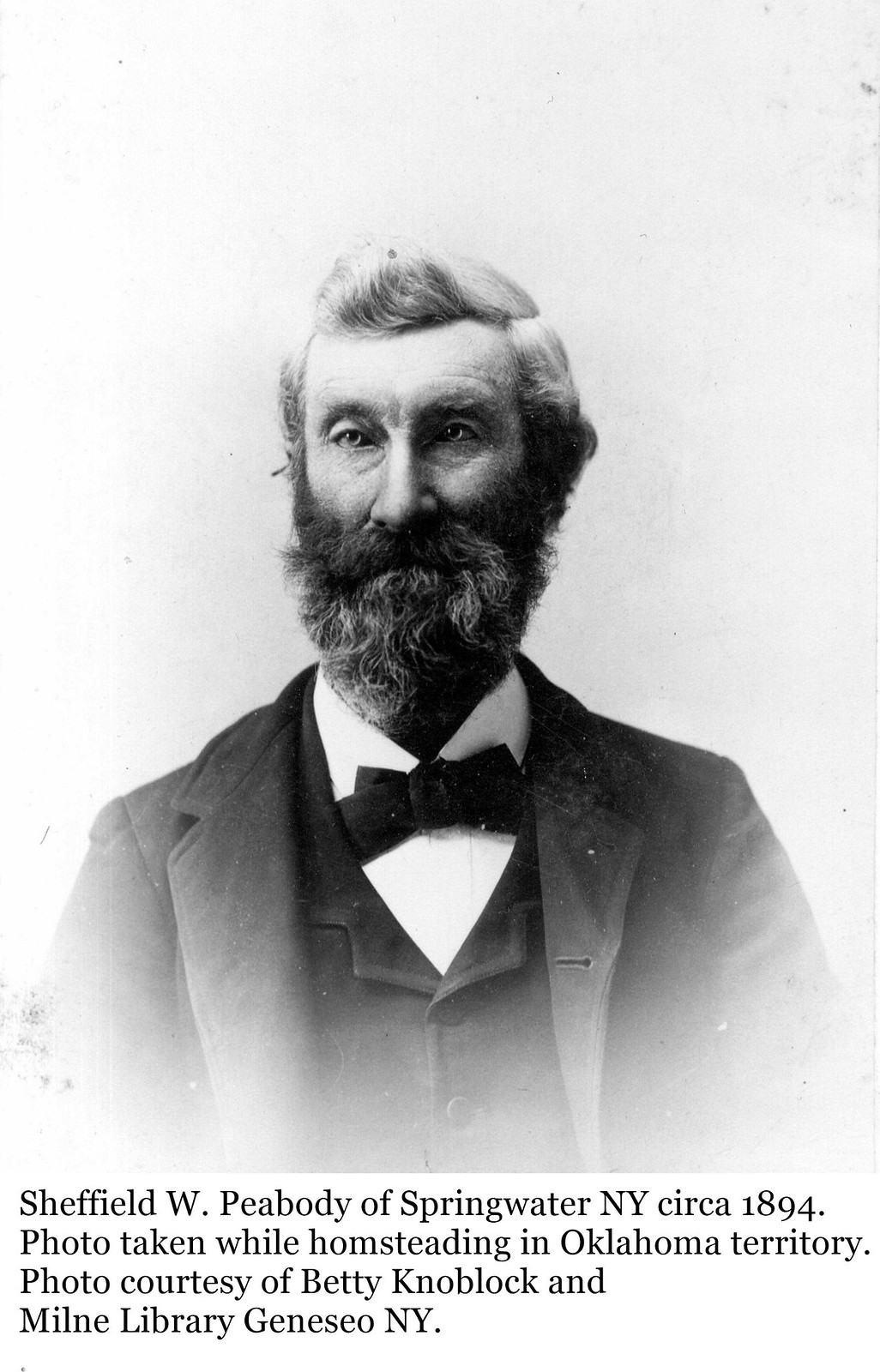This old black-and-white photograph from circa 1894 features a distinguished elderly man, captured from the middle of his chest upwards. He is dressed immaculately in a dark overcoat paired with a white collared shirt and a dark-colored bow tie. His medium-length white hair is neatly combed, and he sports a full beard and mustache, with some gray hairs visible. His facial features include a long nose and beady eyes. The photograph, though showing some dirt marks and fading around the corners, is in pretty good shape, allowing the man's features to be seen clearly. The bottom of the photograph contains a black text caption that reads: "Sheffield WP, body of Springwater, New York circa 1894. Photo taken while homesteading in Oklahoma Territory. Photo courtesy of Betty Knoblock and Milne Library, Geneseo, New York."